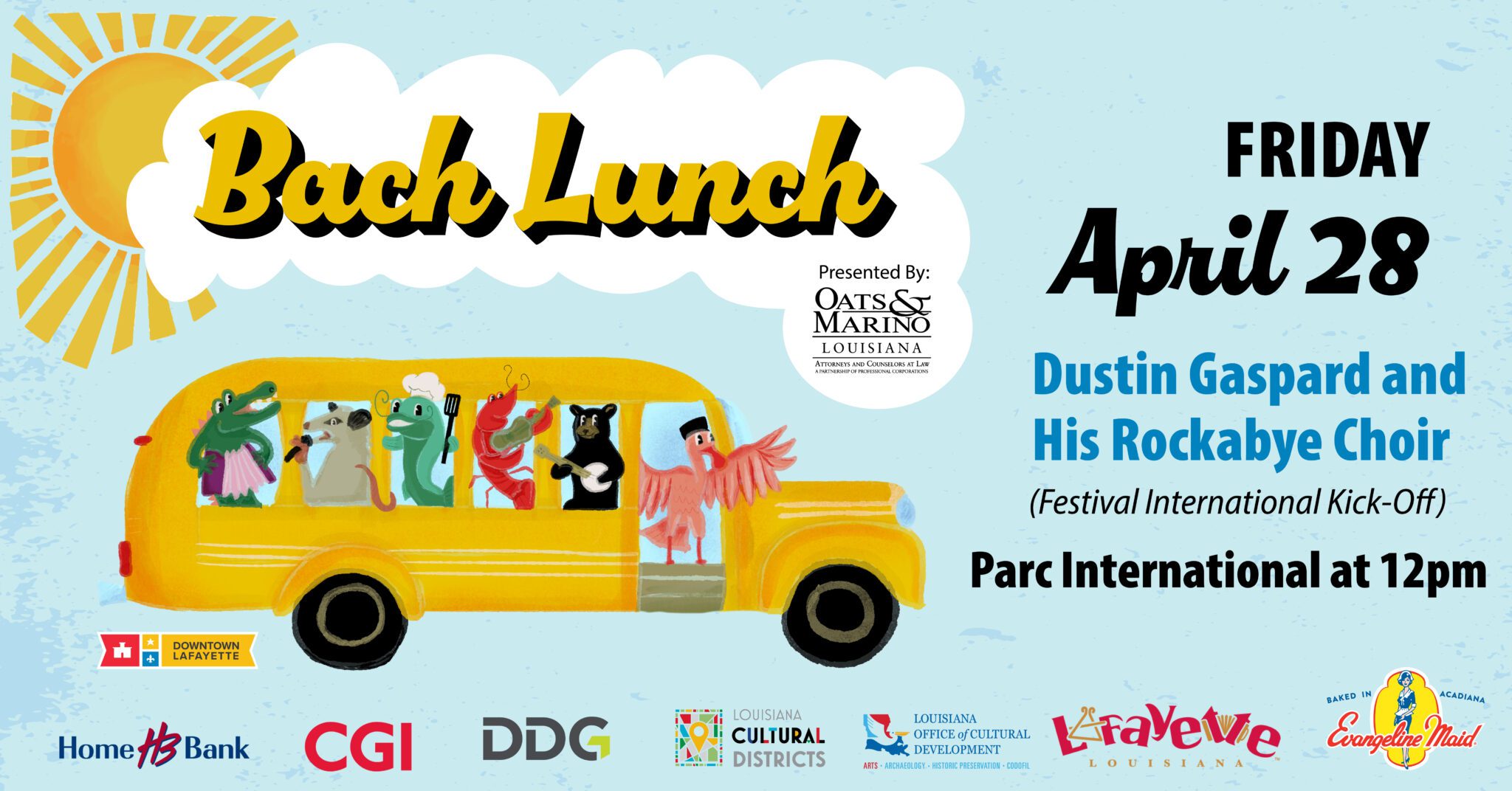This vibrant advertisement showcases a whimsical cartoon illustration of a yellow school bus filled with animated animals, each engaged in various activities. Positioned predominantly in the bottom left, the bus features a pink flamingo at the front, followed by a black bear playing a banjo and a red lobster with a fiddle. Further back, a green fish or dolphin, sporting a chef's hat, holds a spatula, while a possum sings into a microphone, and a crocodile plays an accordion. Above this scene, a white cloud graphic contains the event title, "Bach Lunch," written in large yellow cursive with a black shadow effect, and notes it is "Presented by Oats and Marino, Louisiana." Just above the cloud, a bright yellowish-orange sun with radiating beams adds a cheerful touch. To the right, bold text in black and blue announces, "Friday, April 28th, Dustin Gaspard and his Rockabye Choir," followed by "Festival International Kickoff" and "Parc International at 12 p.m." The light sky blue background further enhances the playful and inviting atmosphere. At the bottom of the image, logos of various sponsors, including Home Bank, CGI, DDC, Louisiana Cultural Districts, Louisiana Office of Cultural Development, Lafayette, Louisiana, and Evangeline Maid, are neatly arranged, adding a touch of formality to this lively and engaging event promotion.